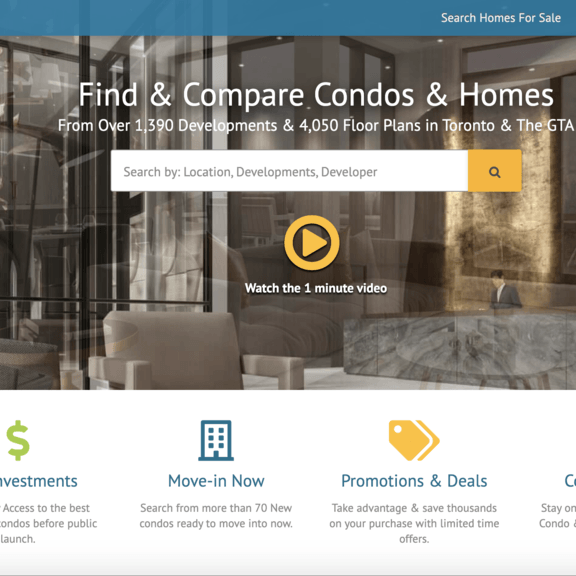The screenshot captures a promotional section from a real estate website. The layout features a stylish theme with a pristine background image of an elegant home. At the top, a prominent line reads, "Search Homes for Sale," inviting users to explore the site. Overlaid onto the background image is a striking white text that encourages potential buyers to "Find and Compare Condos and Homes." Additional information specifies that users can browse through over 1,390 developments and 4,050 floor plans in Toronto and the Greater Toronto Area (GTA).

Directly below the inviting message is a functional search bar, facilitating easy navigation and home searches for users. Beneath the search bar, a call-to-action button prompts visitors to "Watch the one minute video," accompanied by an eye-catching orange video icon.

The lower part of the screenshot, set against a clean white background, extends the advertisement with succinct yet compelling text on the left side. It covers several enticing topics: 
1. **Investments**: Gain access to the best condos before public launch.
2. **Move-in Now**: Search more than 70 new condos ready for immediate occupancy.
3. **Promotions and Deals**: Take advantage and save thousands on your purchase with limited-time offers.

The overall layout is designed to attract potential buyers with its user-friendly interface and focus on exclusive investment opportunities and savings.